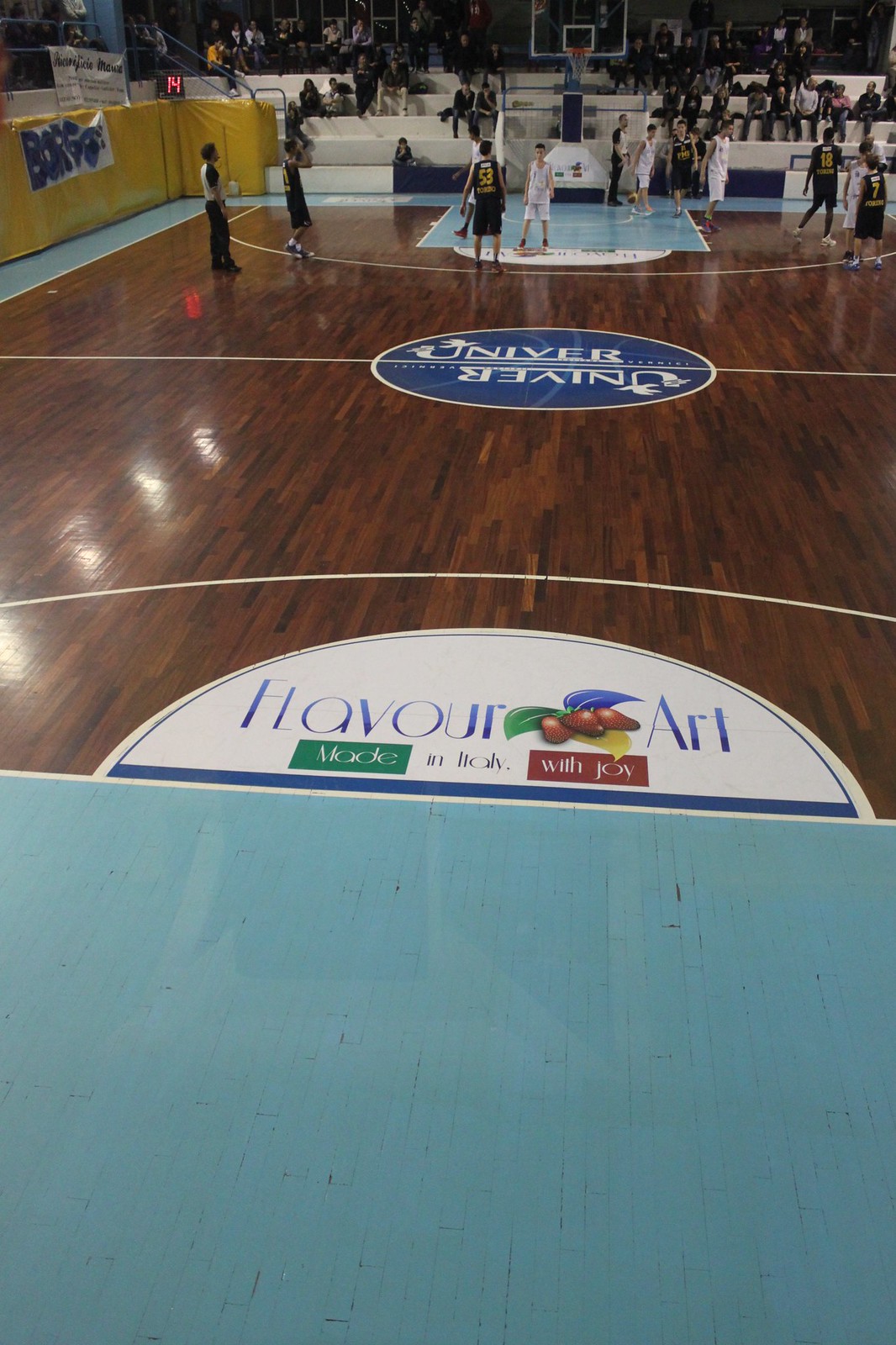The image captures a vibrant basketball game in a well-lit indoor court, taken in portrait orientation. The photograph is viewed from behind a blue wall, obscuring about the lower third of the image. Above this wall, the shiny, dark brown wooden floor of the court emerges. Central to the perspective is the free-throw line, prominently displaying a logo that reads "FLAVOR ART" in blue text with a cluster of fruits, underneath which are the words "Made in Italy with Joy" segmented by green, white, and red boxes. Towards the far end of the court, players in black and white uniforms await the inbound pass under the watchful eyes of referees. The action is halted momentarily, with players poised and ready for the next play. A crowd of 40 to 50 spectators are visible seated in white bleachers behind the hoop, framed by a yellow wall running down the left-hand side of the court. The detailed depiction exudes photographic realism, effectively highlighting the lively atmosphere of the basketball game.